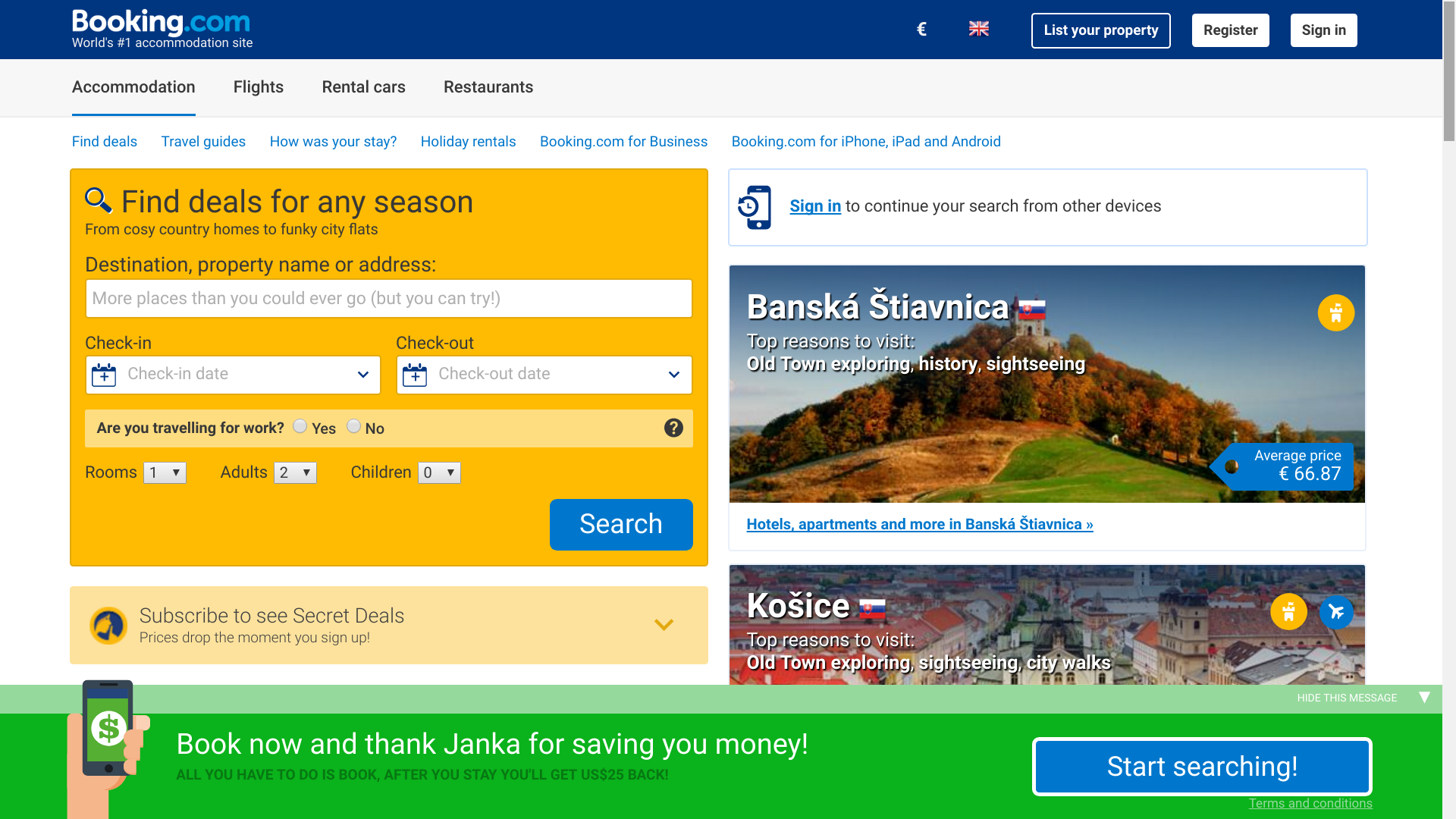This image is a detailed screenshot from the Booking.com website. At the top of the page, there is a navy blue header. On the left side of this header, the Booking.com logo is prominently displayed, with "Booking" written in white font and ".com" in light blue. Beneath the logo, the tagline "World's Number One Accommodation Site" is written in white font. On the right side of the header, there are three clickable options: "List your property," "Register," and "Sign in," each represented by white rectangular buttons.

Below the header, the main section of the website features a white background and four key categories: "Accommodations," "Flights," "Rental Cars," and "Restaurants." Under these categories is a large yellow rectangle with the text "Find deals for any season." This section serves as the search box, containing several white rectangular input fields for users to enter their destination, check-in date, check-out date, and whether they are traveling for work. Additional fields allow users to specify the number of rooms, adults, and children in their party. In the bottom right corner of this yellow box, there is a blue "Search" button.

On the right side of the webpage, a couple of photos are displayed. The top photo is labeled "Banska Stiavnica," showcasing a picturesque hill adorned with beautiful autumn foliage, a green field in the foreground, and a clear blue sky in the background.